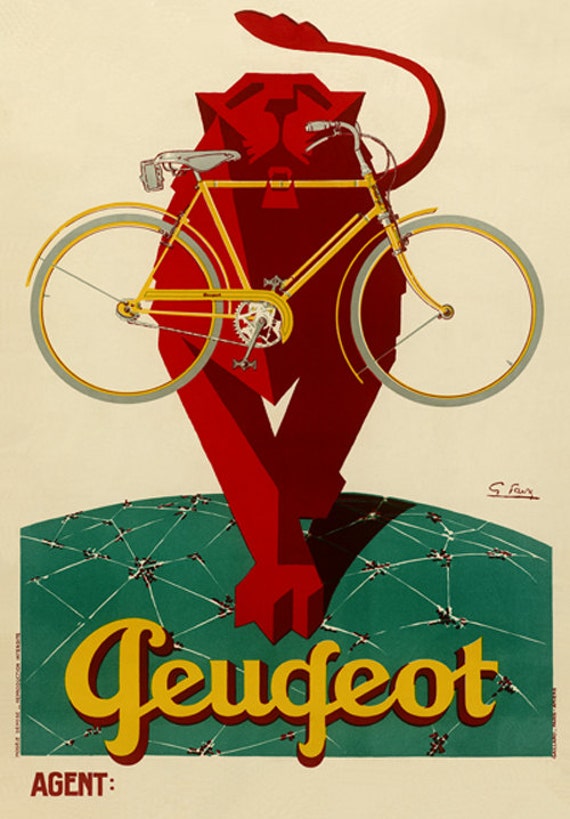This vintage poster portrays an intriguing, retro-style illustration of a large red feline, resembling a lion, with its long tail swinging behind it. The lion is depicted with its mouth open, displaying its fanged teeth, and remarkably, it is holding a yellow bicycle by its fangs. The bicycle features green or blue tires and matching green or blue seat and handlebars. This striking figure stands atop a green half-globe or dome-like structure with white lines, evoking a pattern similar to a spiderweb or a delineated globe. Below this scene, in yellow cursive, are the letters "G-E-U-G-E-O-T," and further down, in red letters, it reads "agent;" suggesting a foreign origin or brand with possible artistic or commercial intent.